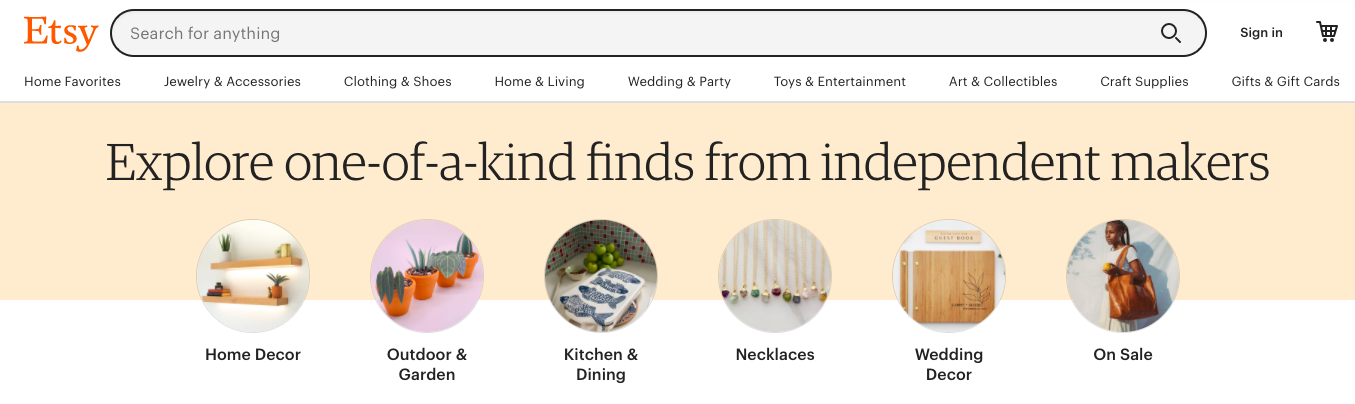This is a detailed screenshot from an Etsy page. The image shows a web page with a white background. In the top left corner, the Etsy logo is prominently displayed in red, followed by a search bar with the placeholder text "Search for anything." Below the search bar, a horizontal menu is visible with category links in black text: Home Favourites, Jewellery and Accessories, Clothing and Shoes, Home and Living, Wedding and Party, Toys and Entertainment, Art and Collectibles, Craft Supplies, and Gifts and Gift Cards. On the right side of the menu, there are two options: Sign In and Cart.

Just below this menu, a pale yellow banner spans the width of the screen. The banner features black text that reads, “Explore one of a kind. Find some independent makers.” The lower half of the screenshot showcases six circular images partially overlapping the yellow banner, with the lower part of the circles extending into a white band.

1. The first circle is labeled "Home Decor" and shows shelves adorned with decorative items, including a couple of plants.
2. The second circle is labeled "Outdoor and Garden" and depicts a diagonal line of plants in terracotta pots against a purple background.
3. The third circle is labeled "Kitchen and Dining," featuring an image with blue fish patterns—likely on a tablecloth or dishcloth—with some fruit, green elements, and a tiled wall in the background.
4. The fourth circle is labeled "Necklaces," displaying several pendant necklaces in different colors hanging in a line.
5. The fifth circle is labeled "Wedding Decor" and shows a wooden area with a carved plaque above it.
6. The sixth circle is labeled "On Sale" and highlights a black woman wearing a white T-shirt and carrying a large brown leather tote bag over her left shoulder, standing against a grayish wall with her shadow visible on the right.

The screenshot has a unique layout, being wide but not very tall, leading to the need for zooming in to read the smaller text details.